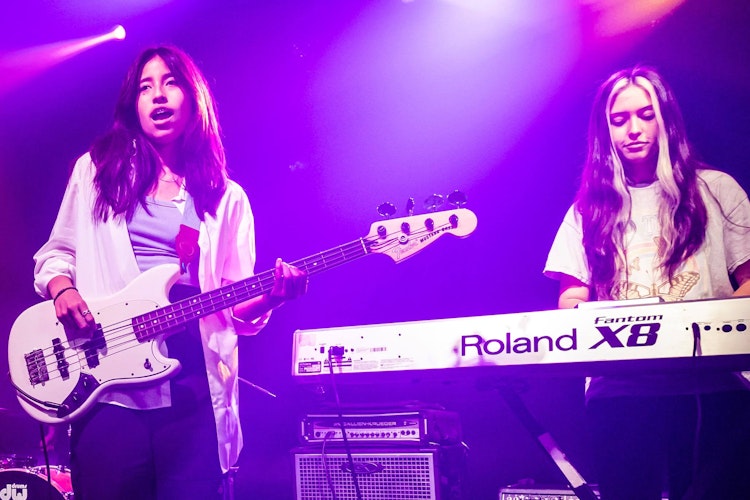This image features two female musicians performing on a stage bathed in purple and pink lighting. The musician on the left, with dark, long hair, is holding a white and black electric guitar and appears to be singing. She is dressed in a white blouse layered over a gray tank top and wears black pants. To her right stands a pianist with long hair, dark with striking white highlights in the bangs. She is focused on playing a Roland X8 Phantom keyboard, which has visible wires extending from its side. The pianist is wearing a white short-sleeved t-shirt with yellow imagery. The atmosphere is vividly colored with spotlights illuminating the performers amidst a backdrop of purple hues.